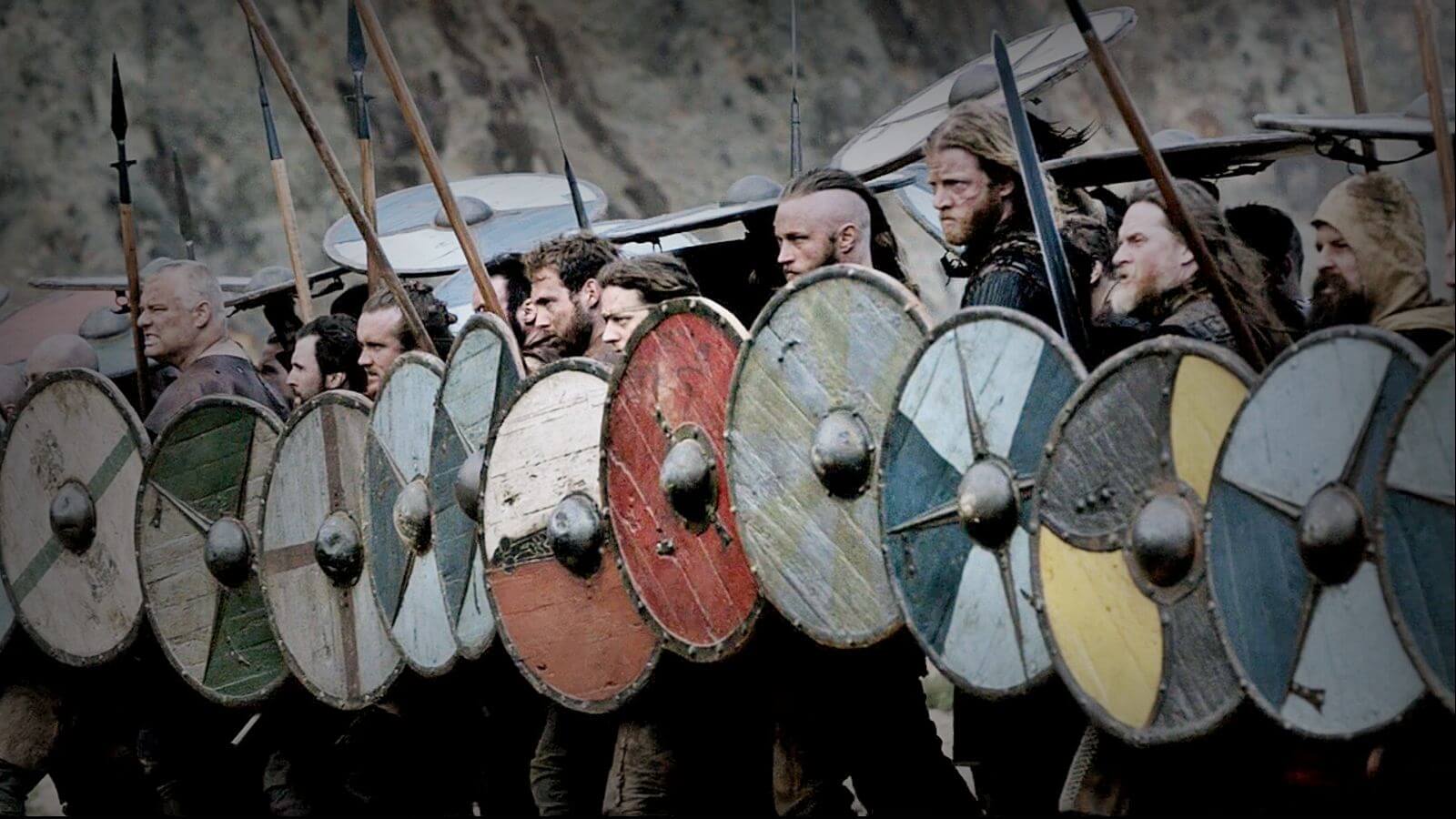In this detailed horizontal color image, likely a still from the popular television series "Vikings" (specifically from season two), a dozen men stand in formation, facing the left side of the frame, ready for battle. Each actor grips a long weapon, either a spear, lance, or sword, and holds a round shield in front of them. The shields, all varying in design and color, include vibrant patterns such as red, green and white, blue and light blue, gray and yellow, and even a half orange and half white shield. The men, many with serious expressions and bearded faces, display distinctive Viking hairstyles, with one notably having his head shaved on the sides and long hair at the back. The backdrop features a grey, rocky hillside with steep terrain, enhancing the historical and rugged atmosphere of the scene.